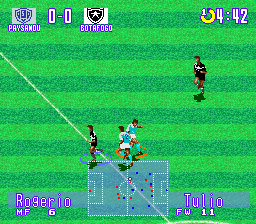This screenshot is from a soccer video game. In the image, there are four players visible on the field. Two of the players are identified with labels indicating their usernames and in-game positions: "Roger_id" who is playing as an MF6 (Midfielder number 6) and "To_Leo" who is designated as FW11 (Forward number 11). The screenshot also captures the game's interface, displaying a timer indicating that there are 4 minutes and 42 seconds left in the match. Below the close-up of the players, the entire soccer field is depicted in a smaller diagram, providing an overview of the players' positions and movements on the pitch. The game's detailed graphical elements and user interface suggest that it is a sophisticated simulation of an actual soccer match.